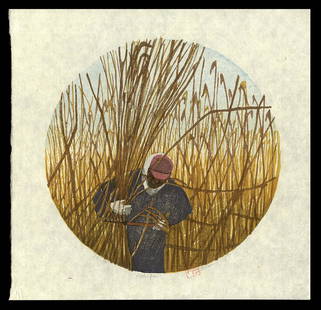The image is a color illustration or painting, likely created with colored pencils, presented in a square format. It features a thick black frame surrounding a beige background with a circular image at its center. This central image depicts a dark-skinned man standing in a wheat field. He is wearing blue overalls, white gloves, a red baseball cap, and holds a sickle in his left hand, appearing to cut the wheat. His right hand is gripping a bundle of tall, dried wheat stalks. The background behind him shows a sky that has a blue-white hue. The man is the main focus, centered within the circle, which is set against a light tan ivory backdrop.